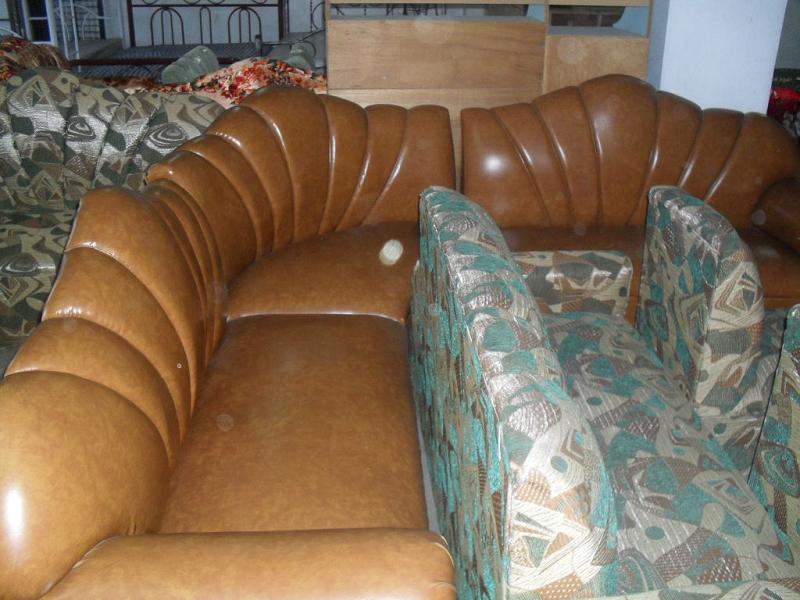This digital photo, taken indoors—likely in a house or a business—depicts a room cluttered with a variety of extremely unattractive couches. Arranged in a tight, almost jumbled manner, the five visible couches appear almost on top of each other, though they are upright and not piled. 

On the far right, there's a hideous loveseat featuring a baffling design with a brown, blue, and gray geometric pattern set against a light green background. In front of this loveseat are two matching chairs that share the same ugly design. Moving leftward, there's a tightly-fitting, shiny faux-leather sectional sofa, curving to the right with a scalloped back and broad armrests, boasting vertical lines. This couch, a very ugly shade of brown, takes up much of the center of the room.

Adjacent to it on the left, another faux-leather couch mirrors its unappealing design. Another prominent piece in the scene is a gold couch with an intricate red pattern, pressed closely against the others. In the background, there are silver bar stools and a black table, along with natural wood shelving units and a white pillar. The overall impression is one of a jumbled storage or sales space, overwhelmed by an array of distasteful and unattractive couches.